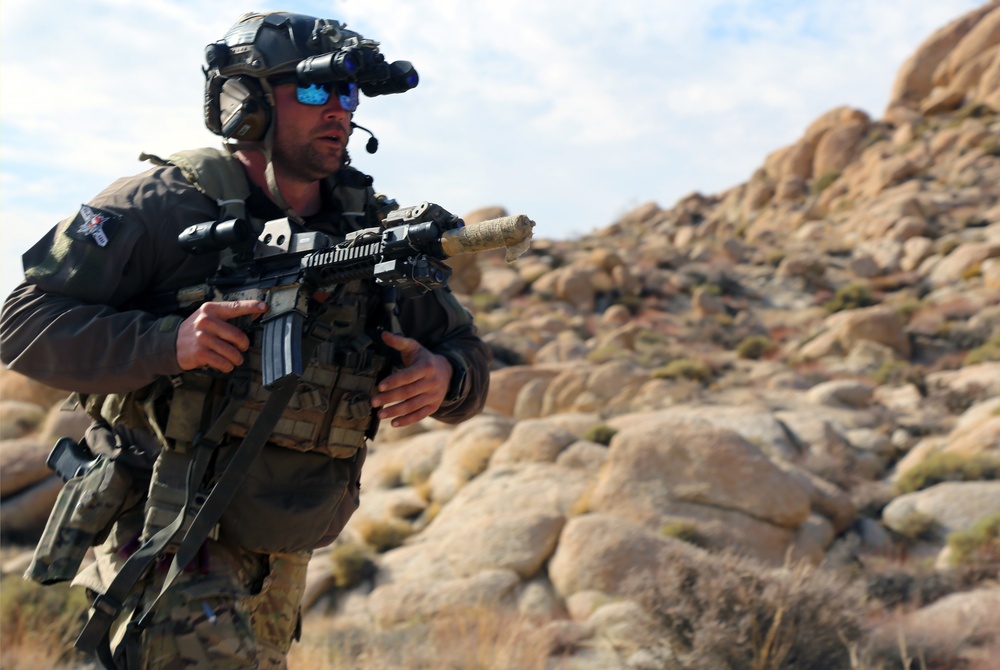This outdoor photograph features a man, likely in the military, positioned on the left side of the frame, visible from the knees up. He sports full army fatigues, including a camo jacket and pants, and a heavy vest. His head is protected by a helmet fitted with a built-in binocular scope, which is currently pulled up on his forehead. He wears reflective blue-lensed sunglasses and has a mic positioned off the side of his face. The man, who exhibits a serious expression with a stubbly beard and mustache, is facing to his right, holding an assault rifle in his left hand, with a pistol holstered on his right hip. The background shows a rugged, desert-like landscape, characterized by a steep accumulation of beige stones and sparse scrubby brush. A light blue sky dotted with white clouds completes the scene, adding to the overall impression of a harsh, arid environment. The photograph captures him mid-motion, suggesting a sense of action and readiness.